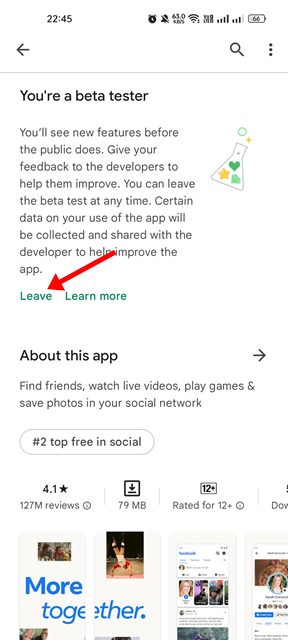In this screenshot, viewed against a white background, we see a detailed interface of a cell phone screen. At the top, the header displays the current time at 22:45 on the upper left. To the right of the time, several status icons are visible: an alarm clock icon, indicating alarms are set; notification settings showing notifications are off; a Wi-Fi symbol indicating Wi-Fi is on; a reception icon showing full signal strength; and a battery icon showing the battery at 66% charge. Below the battery icon, there is a magnifying glass symbol followed by a vertical ellipsis (three dark gray dots arranged vertically).

Directly beneath a light gray horizontal line, bold dark gray text reads: "You're a beta tester." Below this, light gray text provides additional information about the beta program: "You'll see new features before the public does. Give your feedback to the developers to help them improve. You can leave the beta test at any time. Certain data on your use of the app will be collected and shared with the developer to help improve the app."

At the bottom, there are action buttons in green text: "Leave" and "Learn more."

In the upper right corner, there is an illustration combining green, yellow, and gray colors, featuring a test tube bottle adorned with a heart and a star, symbolizing the beta testing phase.